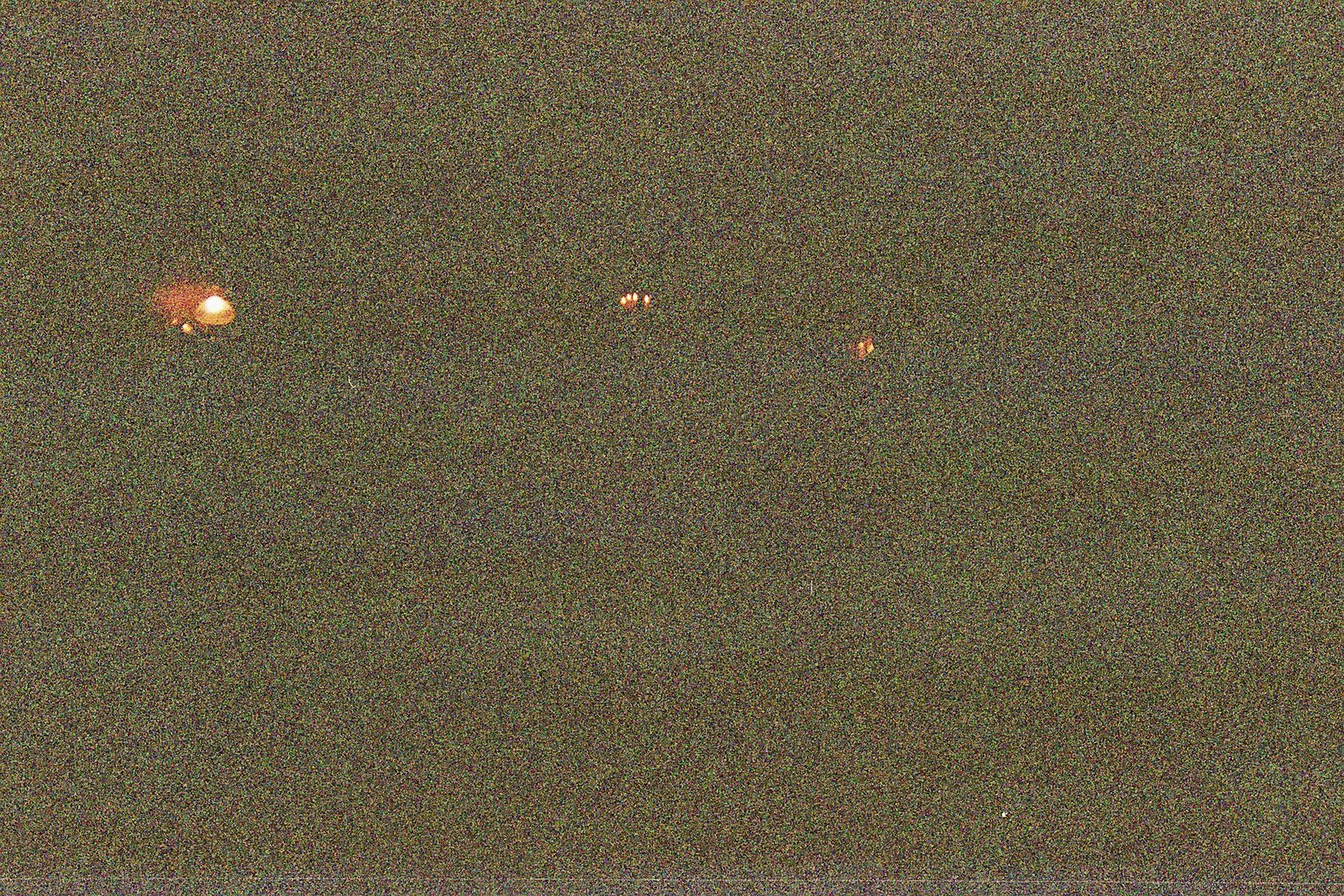The image depicts a dark, pixelated background that appears to have been photographed in low light. This background, a mix of patchy green and dark tones resembling a night sky or a poorly lit room, features three distinct light sources. On the upper left, there is a large, dome-shaped structure reminiscent of a mushroom or an onion lamp, with a metal brown stem. This structure glows orange around the edges and transitions from yellow at the base to white at the top due to the illumination from its bulb, casting an orangey glow around it. Closer to this dome-shaped light are two small white dots surrounded by an orange hue. In the center of the image, there is another irregularly shaped orange light with four white pinhole-sized dots arranged in a clustered pattern. Finally, towards the right side, there are two small white dots within an orange blur, producing an orange aura. The three lights vary in size and intensity, transitioning from the largest and most complex on the left to the smaller, simpler lights on the right.